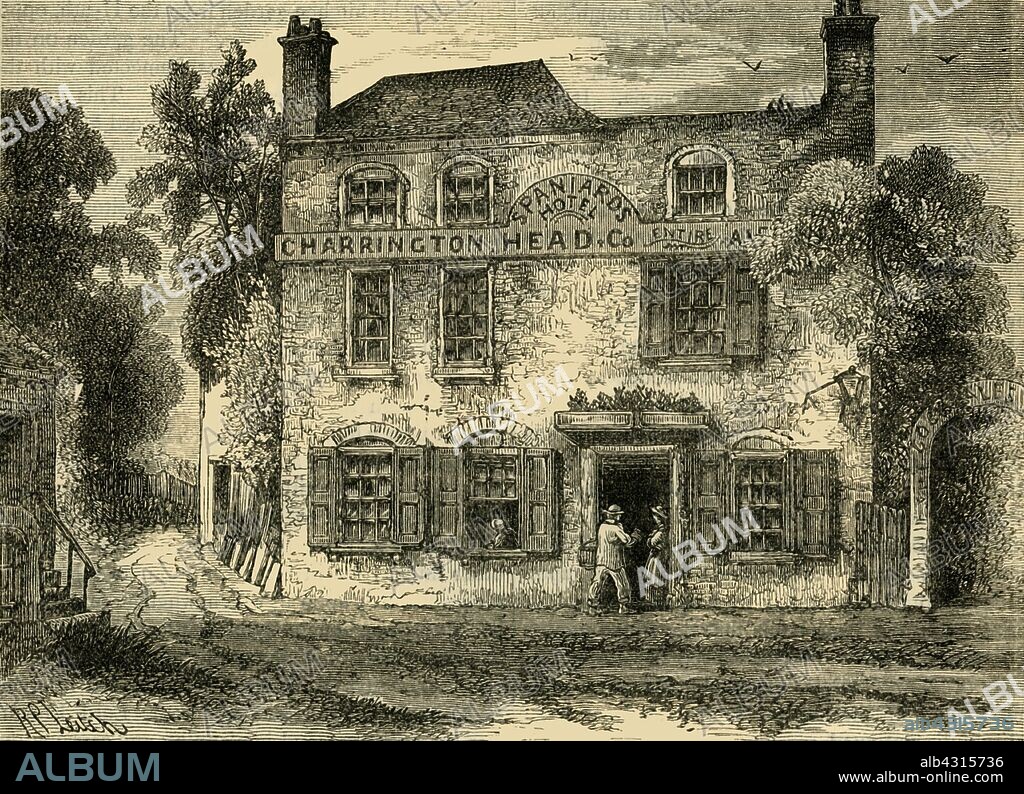This image features a scanned drawing sourced from an old newspaper or historical artist's work. It has watermarks diagonally imprinted with the word "album," accompanied by a black border at the bottom, which also reads "album." Additionally, the bottom right corner bears the URL "www.album-online.com" along with a serial number, suggesting where the image might be obtained without the watermark. The drawing itself, styled reminiscent of illustrations found on dollar bills, features a sepia tone rather than stark black and white coloration.

At the center of the image is a historic building labeled "Charrington Head & Co., Spaniards Hotel," indicating its current use as a residence or lodging. The building showcases architectural details, including two chimneys, one on each end, and six window panes, one of which is ajar, revealing an occupant inside. The scene includes two or three figures entering the building, enhancing its narrative of daily life.

To the right of the building, a tree, an arched entrance gate, and a portion of the pathway add to the picturesque setting. On the left, more trees, an additional path leading to the side of the building, and a partially visible outbuilding contribute further depth and context. The artist's initials, "R.P.," are inscribed at the bottom of the image, marking their work.

Overall, this detailed depiction captures a moment in time, providing a window into the past and the everyday existence surrounding the Spaniards Hotel.